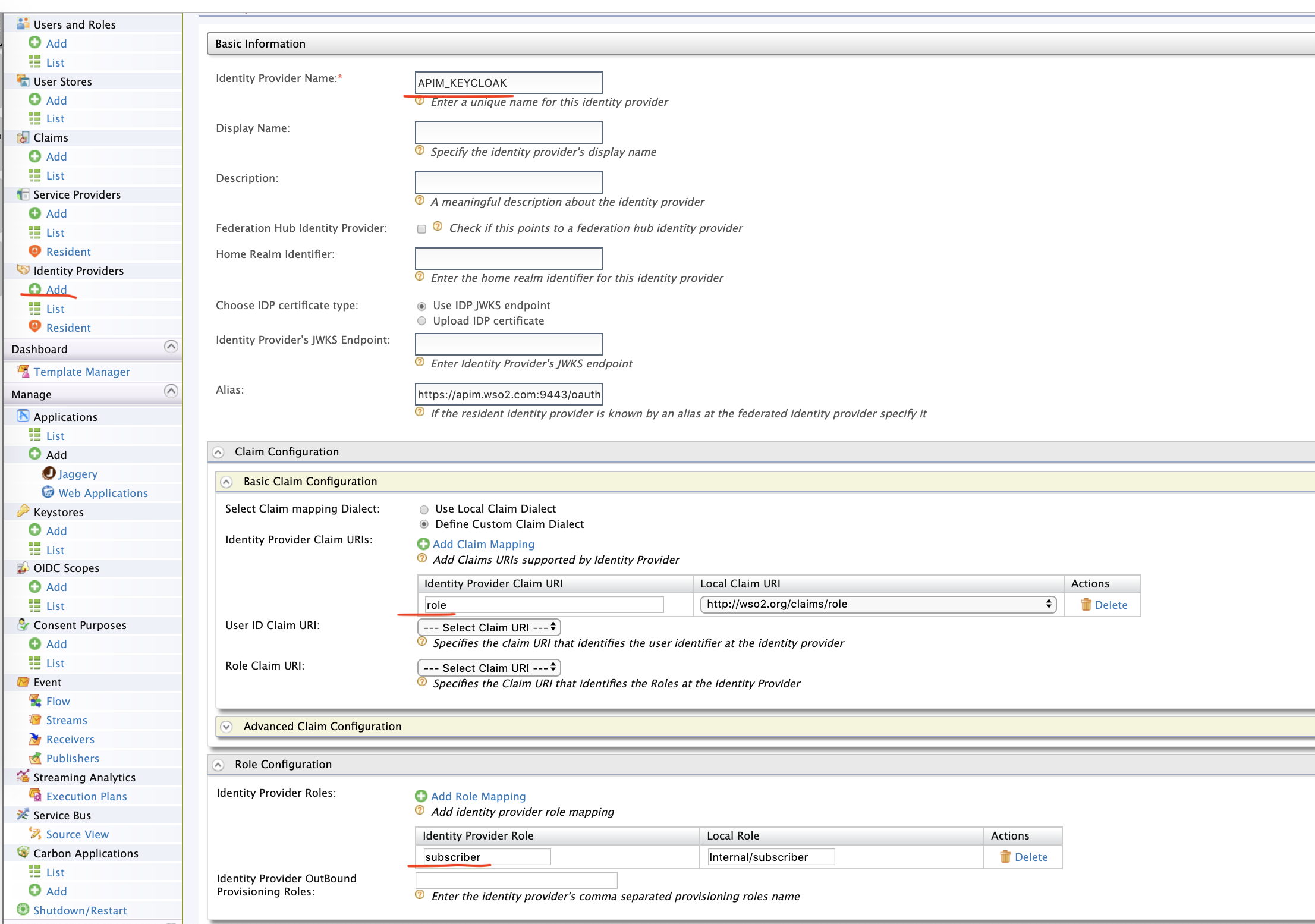The image depicts a comprehensive software interface, likely a web-based administrative portal, designed to manage various configurations. The user interface has a vertical navigation bar on the left side. This navigation bar contains multiple sections including "User Roles" (with options to add and list them), "User Stores" (with options to add and list), "Claim Providers" (featuring options to add, list, or manage residents), and "Identity Providers" (also with add, list, or resident management options). "Add" buttons in these sections are highlighted in red, drawing attention to the option to create new entries.

To the right of the navigation bar, a panel entitled "Basic Information" is visible, where users can input the "Identity Provider Name." In the current context, the name entered is "apim_keycloak," with the entry underlined in red to indicate importance or error.

Other prominent sections visible in the interface include "Dashboard," "Manage Applications," "Keystones," and several configuration settings such as "Basic Claim Configuration," "Advanced Claim Configuration," and "Role Configuration." Within the "Basic Claim Configuration" section, the term "role" is underlined, while in the "Role Configuration" section, the word "subscriber" is similarly marked.

The interface predominantly uses a white background, with text primarily in blue and black, facilitating readability. The red underlines and highlights emphasize critical fields and options that require user attention. The overall layout is dense, suggesting a powerful, feature-rich platform intended for users who require detailed control over various administrative and identity-related aspects.

This image likely serves as a guide or tutorial, showing users how to navigate and utilize this intricate software for managing configurations on the platform.